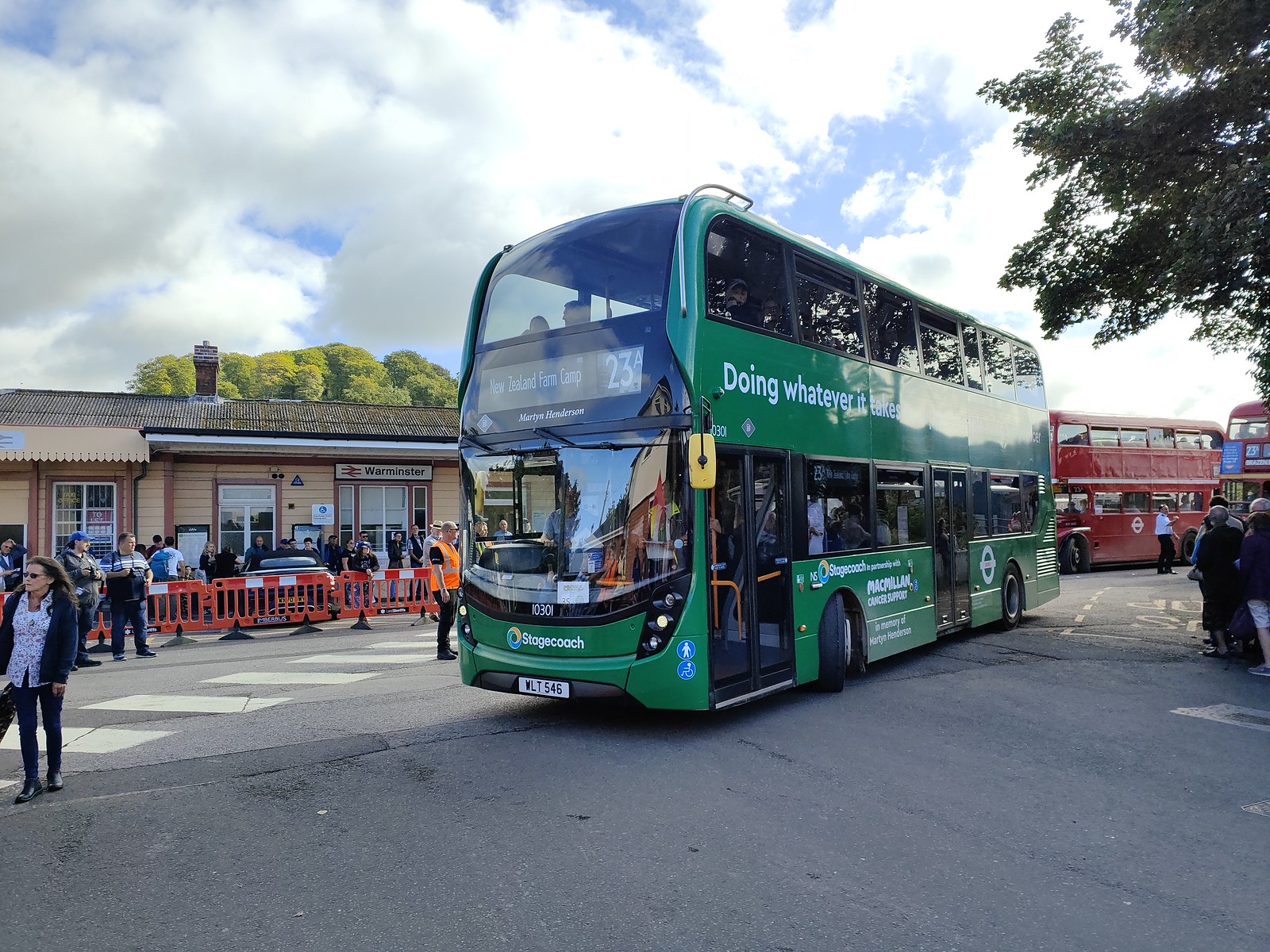The photograph, taken on a bustling city street during the daytime, prominently features a green double-decker bus operated by Stagecoach, numbered 23A, and adorned with the partially visible slogan "doing whatever." The bus is caught in motion, heading towards the viewer, preparing to make a stop where a large crowd awaits behind an orange barricade. The crowd includes people waiting to board, as well as a man in an orange vest who seems to be directing traffic. Among the crowd, a woman dressed in a long black sleeve sweater, black pants, a white shirt, and sunglasses walks toward the camera on a white crosswalk. In the background, a long, peach-colored building labeled "Warminster" stands under a blue sky filled with thick, white clouds. Two more double-decker buses, both red, are situated behind the green bus, adding to the bustling scene. The pavement is marked with gray tarmac and white rectangles for crossing, further indicating the street's busy nature.